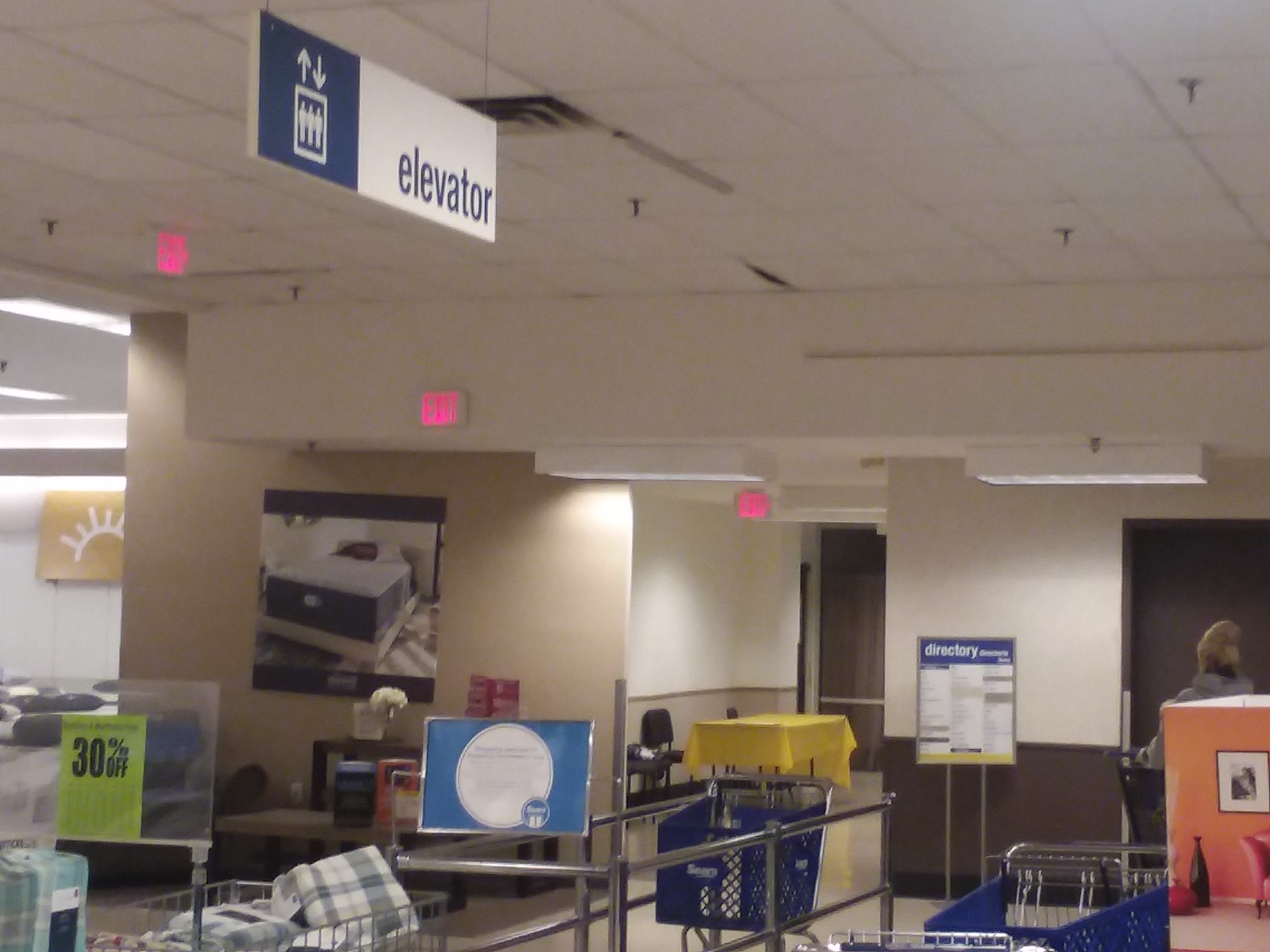The image captures the interior of a room, which appears to be part of a grocery store. The ceiling is adorned with white, squared tiles. A prominent sign hangs down from the ceiling. The left side of the sign is blue, featuring a white symbol of three figures and arrows pointing upward and downward, indicating elevator directions. The right side of the sign is white with the word "Elevator" inscribed in blue.

On the walls, several pictures and posters are visible. To the left, there is a yellow rectangular poster with a simple white drawing of a sun. Facing directly forward is another rectangular poster. Adjacent to these, a bright green rectangular sign prominently displays "30% off." Nearby, a smaller blue sign can be seen.

In the foreground, there are two blue shopping carts. In the background, a table covered with a yellow tablecloth is visible, and a sign labeled "Directory" is positioned towards the front of the image. Further to the right, there is a noticeable orange square, possibly another signage or decoration. The space is well-organized and visually informative, guiding customers effectively through various cues and signs.